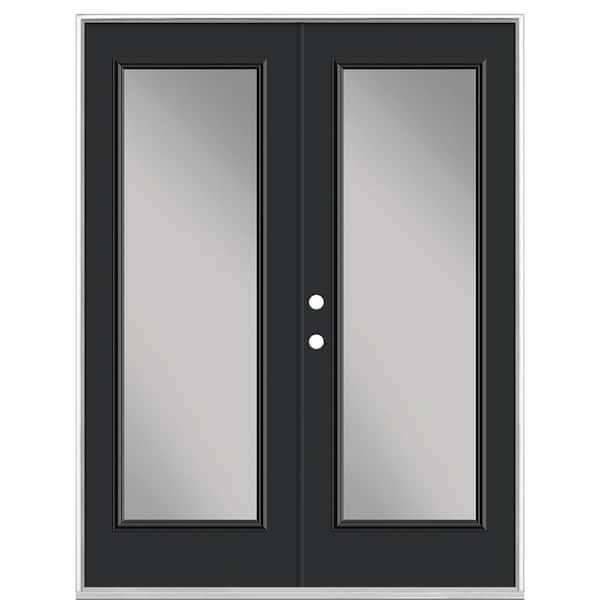The image is in portrait orientation and features a tall, double-panel black door set against a contrasting light border. Each door panel is fitted with large rectangular glass windows that have a muted, light gray appearance, possibly due to a film that obscures transparency. In the middle of the right-hand door panel, there are two small white circles that appear to be the door handle and lock. The frame of the doors is distinctly black or dark gray, accentuated by the lighter bordering frame which enhances the overall starkness and simplicity of the composition. The image leaves an impression of minimalist design, capturing the essence of a functional yet modern entrance.